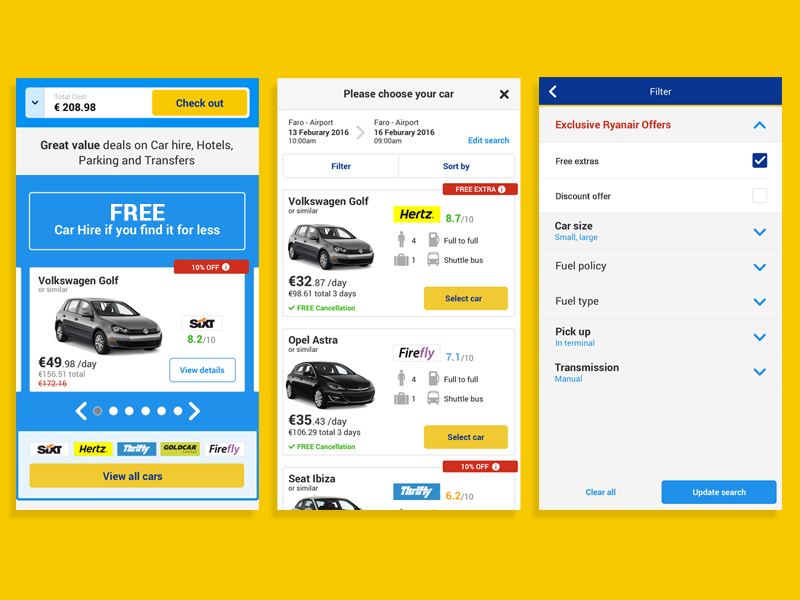### Detailed Caption:

The images display a series of screenshots from a mobile application, the specific platform of which is not identifiable due to the clipped nature of the images. These screenshots appear to belong to a rental car application. 

---

#### Screenshot 1:
This screenshot features the checkout screen of a rental car booking system. 

- **Header:** At the top, there's a bar that displays the total cost of the rental, which is €208.98. Adjacent to this, a prominent yellow button labeled "Checkout" is visible.
- **Promotional Banner:** Below the header, a gray banner is situated on a light blue background, reading "Great value deals on car hire, hotels, parking, and transfers."
- **Offer Summary:** The main content area has a white rectangle against the blue background. Within it, white text declares, "Free car hire if you find it for less."
- **Car Offer:** The offer features a Volkswagen Golf or a similar vehicle, highlighted with a red banner indicating "10% off." It is priced at €49.98 per day, amounting to a total of €156.51. There is a "View Details" button for this offer.
- **Agency & Rating:** Above the car offer, the rental agency's logo, which seems to be "SIXT," is displayed. Below that, a rating of 8.2 out of 10 is provided.
- **Scrolling Element:** At the bottom, there’s a horizontal scrolling element indicated by carets pointing left and right and eight white dots, signifying multiple offers available for browsing.

---

#### Screenshot 2:
The central screenshot highlights the car selection process.

- **Header:** "Please choose your car" is displayed at the top, alongside the rental period details—pickup at Faro Airport from 13 February 2016, 10 a.m., to 16 February 2016, 9 a.m.
- **Filtering Options:** There are buttons for "Filter" and "Sort by."
- **Car Listing:**
  - **Volkswagen Golf Offer:** Priced at €32.87 per day, totaling €98.61 for three days. This offer is from Hertz and features a rating of 8.7 out of 10. A red banner labeled "Free extra" is also visible.
    - **Details:** The vehicle accommodates four people, has a gas tank full-to-full policy, holds one bag, and includes a shuttle bus service. It also offers free cancellation, marked by a green check mark.
  - **Additional Offers:** Beneath the Volkswagen Golf, there are listings for an Opel Astra from Firefly and a Seat Ibiza from Thrifty.

---

#### Screenshot 3:
The final screenshot details the filter options for refining search results.

- **Header:** A red banner at the top announces "Exclusive Ryanair offers."
- **Filter Options:** Several filter options are presented.
  - **Free Extras:** This option is checked.
  - **Discount Offer:** This option is not checked.
  - **Car Size:** Options for small and large are visible.
  - **Fuel Policy and Type:** These fields are currently unselected.
  - **Pickup Location:** In-terminal option is chosen.
  - **Transmission:** Manual is selected.
- **Actions:** At the bottom, "Clear All" and "Update Search" buttons are available for refining or resetting the search criteria.

---

This detailed caption provides a comprehensive description of the screenshots, preserving the specifics and contextual information provided.